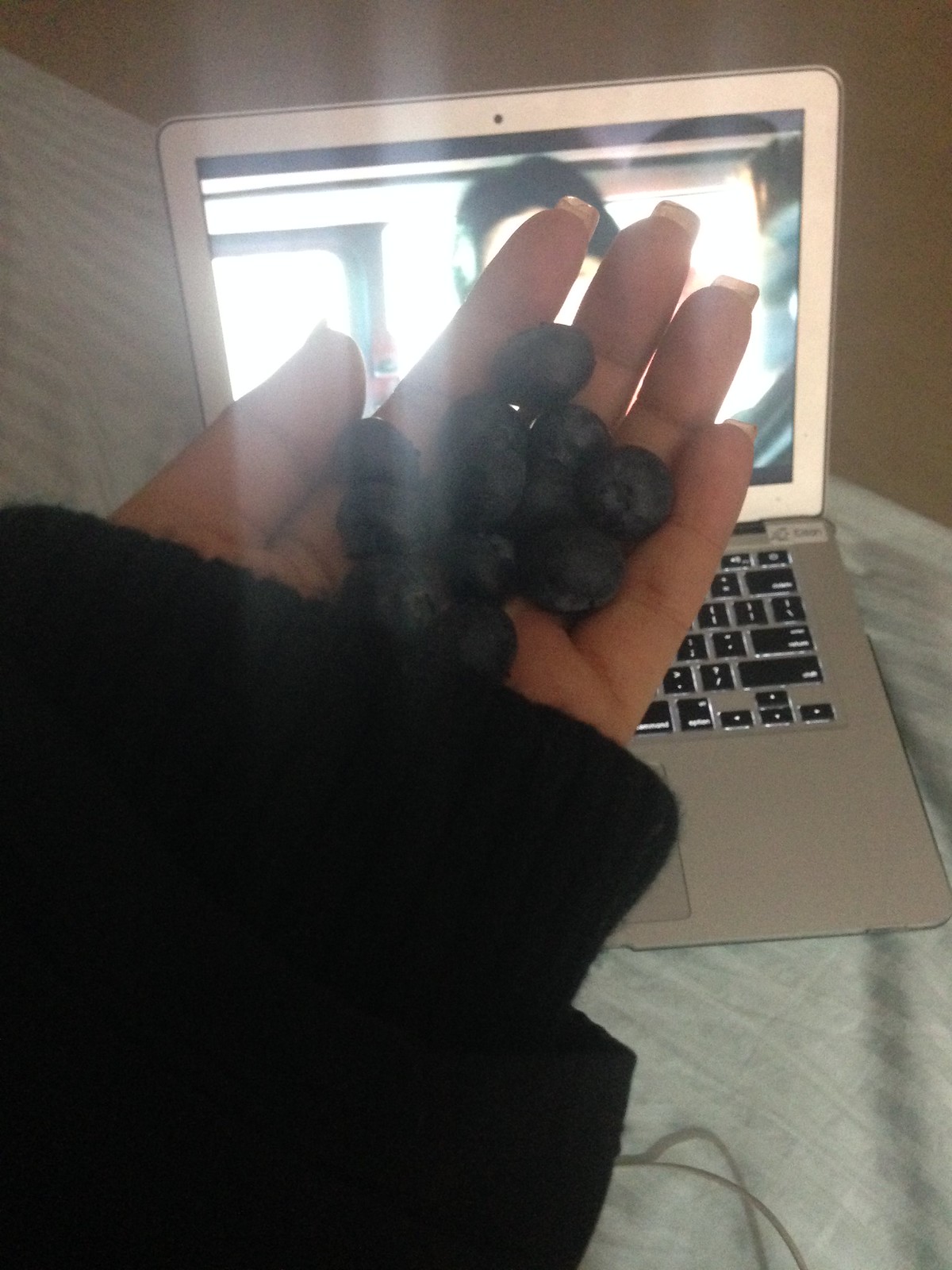In this photograph, a female hand with long, squared-off fingernails is holding approximately 12 blueberries. The hand is emerging from the sleeve of a black jacket or a wool sweater that covers up to the palm. This hand and the garment take up most of the foreground. In the background, there is an Apple laptop with a bright display, possibly showing a video that includes a human face. The laptop rests on a bedspread adorned with light gray and green stripes. The setting appears to be inside a room with a tan floor visible in the background. The lighting from the laptop's screen causes a slight blur in the image, casting a soft glow over the scene.